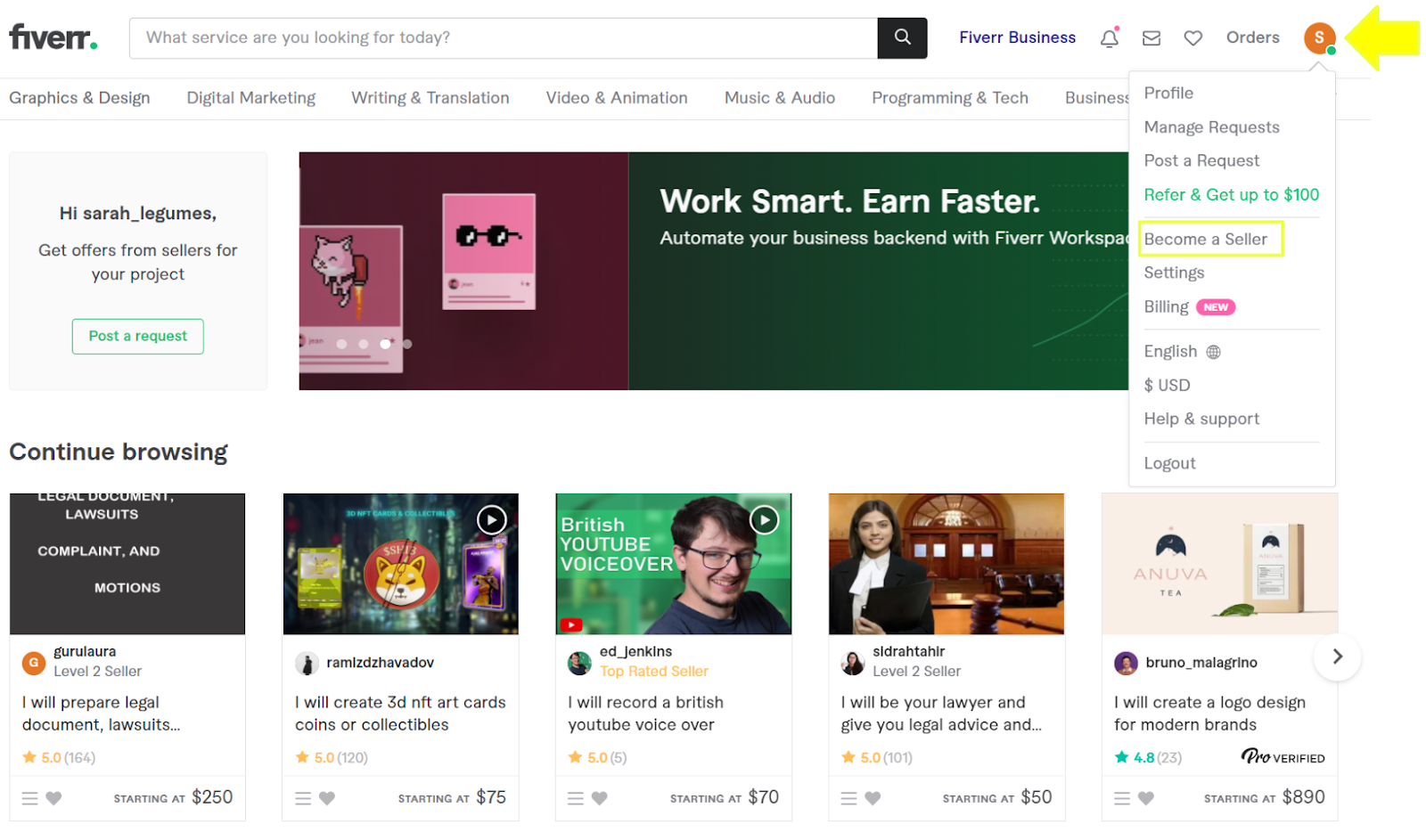This landscape mode screenshot features the Fiverr website interface. In the upper left corner, the Fiverr logo is prominently displayed. Adjacent to it, there is a search bar with a prompt that reads "What service are you looking for today?" accompanied by a magnifying glass icon. To the right of the search bar, various options are visible: "Fiverr Business," followed by a bell icon with a red notification dot, an envelope icon, a heart icon, the word "Orders," and an orange circle containing an 'S' highlighted by a yellow arrow.

Below this navigation bar, several category tabs are lined up, including "Graphics & Design," "Digital Marketing," "Writing & Translation," "Video & Animation," "Music & Audio," "Programming & Tech," and the partially cropped "Business." Additionally, a drop-down menu reveals further options: "Profile," "Manage Requests," "Post a Request," a green-highlighted "Refer and get up to $100," a yellow-outlined "Become a Seller," "Settings," "Billing" labeled as new, "English," "US Dollars," "Help & Support," and "Log Out."

A narrow promotional box beneath this menu reads, "Work Smart, Earn Faster. Automate your business back end with Fiverr Workspace." To its left, a greeting message shows, "Hi Sarah_leggings, get offers from sellers for your project," followed by a green-outlined button labeled "Post a Request."

At the bottom, there is a prompt stating "Continue Browsing," accompanied by several rectangular thumbnail images of different services available on Fiverr.